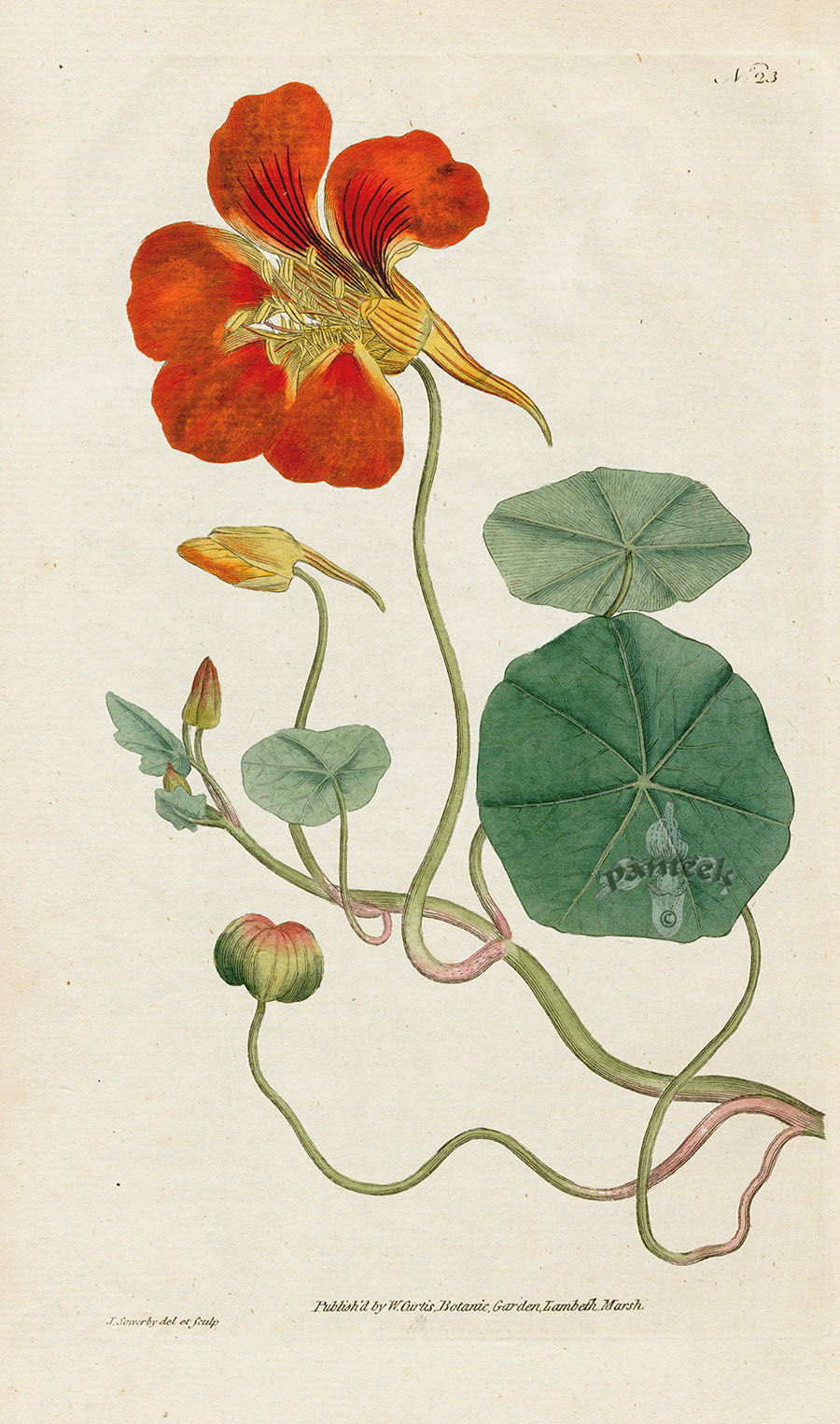This painting features a striking array of botanical elements against a beige, antique-like background. Central to the composition is a winding vine originating from the bottom right of the image, leading up to a stunning, red flower with five petals. The flower, resembling a honeysuckle, blooms vibrantly at the top of the image and is detailed with yellow pistils or stamens at its center. The petals transition from red at the top to yellow at the base.

Further accentuating the painting are multiple smaller branches and vines that extend out from the main one. These branches support several green lily pads—three in total, with one larger and darker and the other two being lighter in color. Along these vines, other green leaves and unblossomed flower buds can be observed.

Additionally, there is a faint watermark with the name “Pammy” in gray located on the largest lily pad. At the very bottom of the image, one can find delicate calligraphy in black, tiny script, difficult to decipher, situated in the left-hand corner and extending slightly towards the center.

Overall, the composition elegantly blends various shades of green leaves, red and yellow hues of the flower, and subtle textual elements, creating a harmonious and detailed botanical artwork.